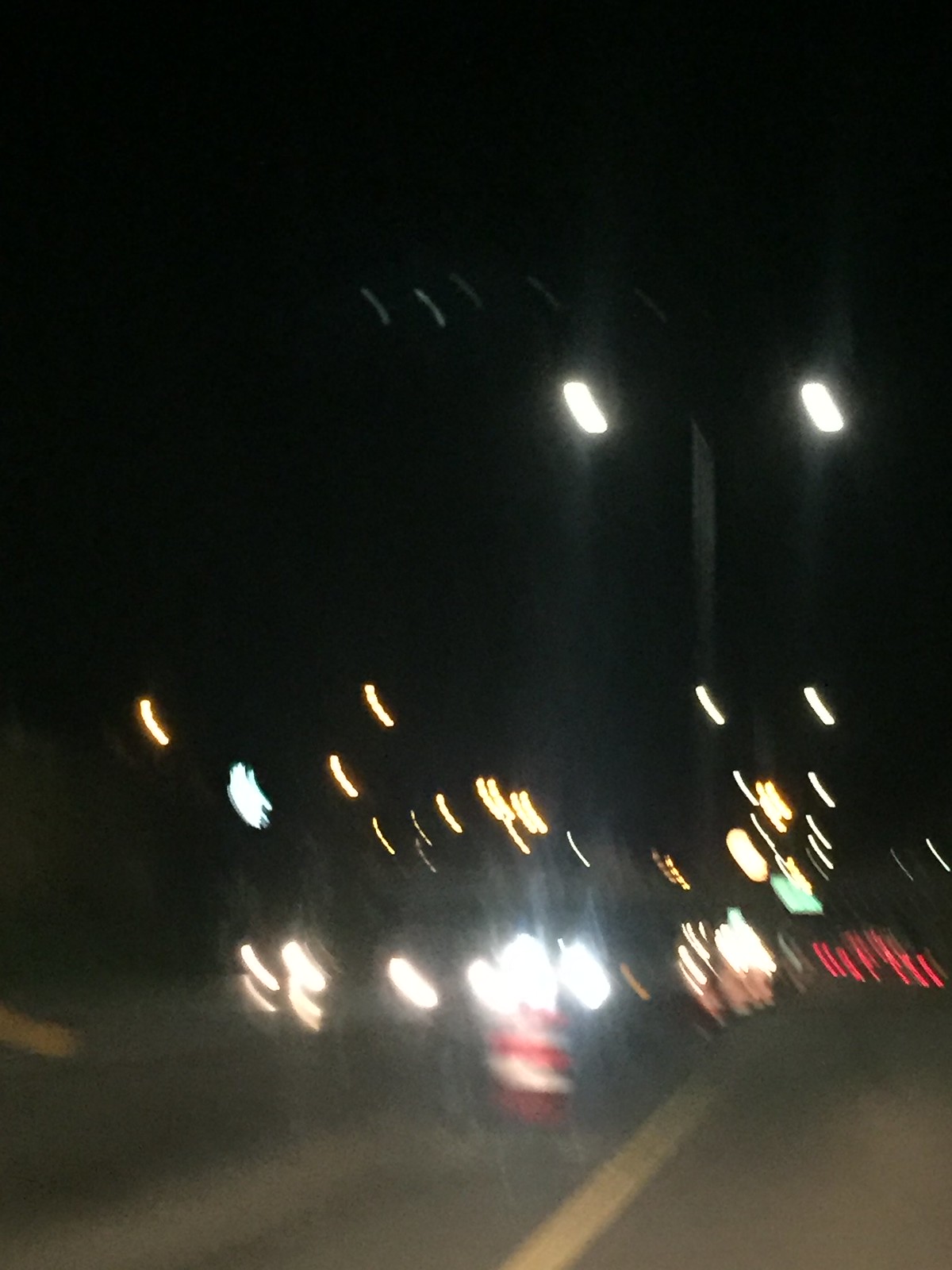A blurry, nighttime shot taken from a moving car, devoid of the vehicle's interior. The image is chaotic from the motion, streaked with a multitude of colorful lights from passing headlights, taillights, and streetlights. Predominantly yellow and white, with occasional hues of blue and red, these lights create an almost abstract, kaleidoscopic effect across the frame. In the lower center, amidst the vibrant light trails, a traffic cone with red and white stripes is faintly discernible. The sky is pitch black, a stark contrast to the bright streaks, emphasizing the low quality of the image and the immediate intensity of the light sources.